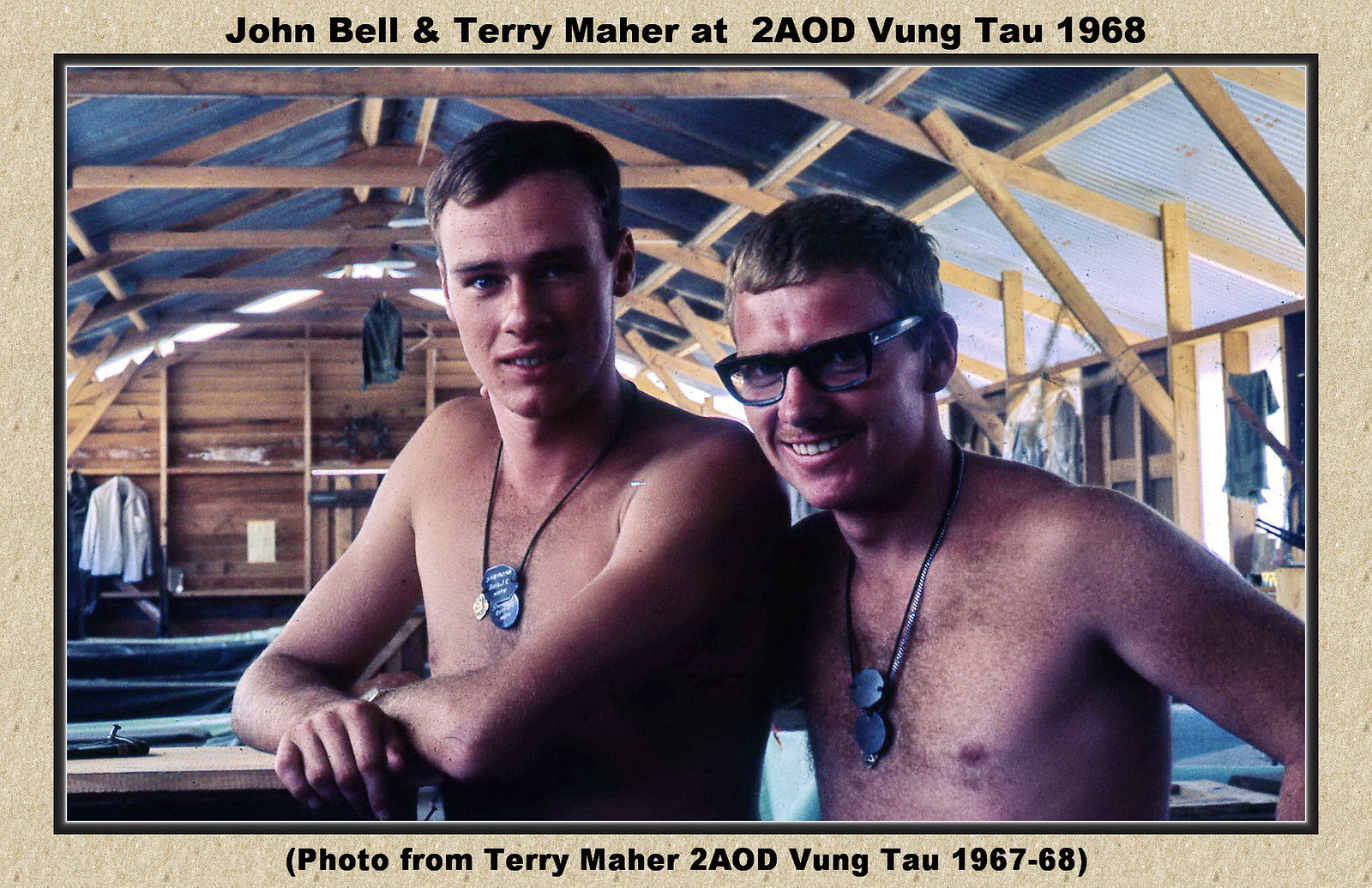The image depicts a horizontal rectangular postcard-style frame on a medium tan background with black text at the top that reads, "John Bell and Terry Maher at 2AOD Vung Tau, 1968". At the bottom, a caption in parentheses reads, "photo from Terry Maher, 2AOD Vung Tau, 1967-68." Within the frame, there's a photograph of two young men, possibly in their late teens or early 20s, both shirtless and wearing military dog tags. They have short brown hair, with the man on the right donning glasses. They stand at a slight angle, with their bodies facing to the right but their heads looking directly at the camera, smiling faintly. The photo is set inside a military barracks, characterized by a wooden frame structure, visible wooden canopy, and possibly a metal roof. In the background, one can see cots and a white shirt hanging on the left. The rustic simplicity of their surroundings, along with their attire, suggests a military installation in Vung Tau during the late 1960s.